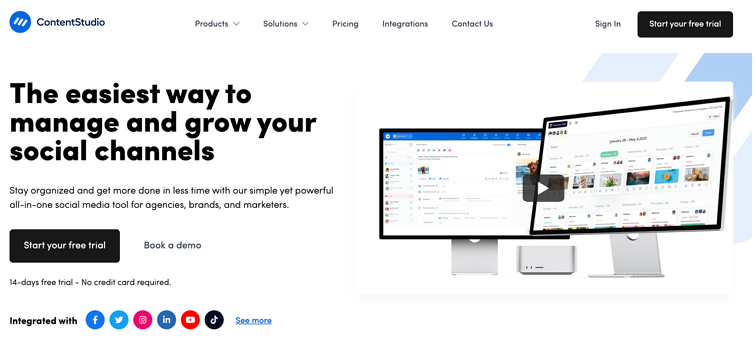The image features a light blue background with a prominent blue circle at the top center, emblazoned with three white lines and the text "Content Studio." Below this circle, a navigation bar includes links to "Products," "Solutions," "Pricing," "Integrations," "Contact Us," and "Sign In."

A striking black box towards the upper section reads, "Start Your Free Trial." Beneath it, bold text proclaims, "The Easiest Way to Manage and Grow Your Social Channels," followed by the tagline, "Stay organized and get more done in less time with our simple yet powerful all-in-one social media tool for agencies, brands, and marketers." Next, another black button offers an invitation to "Start Your Free Trial."

Additional details include a smaller text line: "Book a demo, 14-days free trial, no credit card required." The image showcases integrations with various social media platforms including Facebook and Twitter, highlighted at the bottom with an option to "See More."

On the right side, the image displays two computer screens. One screen shows a series of four or five pictures displayed horizontally. A prominent black square on this screen has a white arrow pointing to the right. Various other computer components are faintly visible in the background, adding to the technical ambiance.